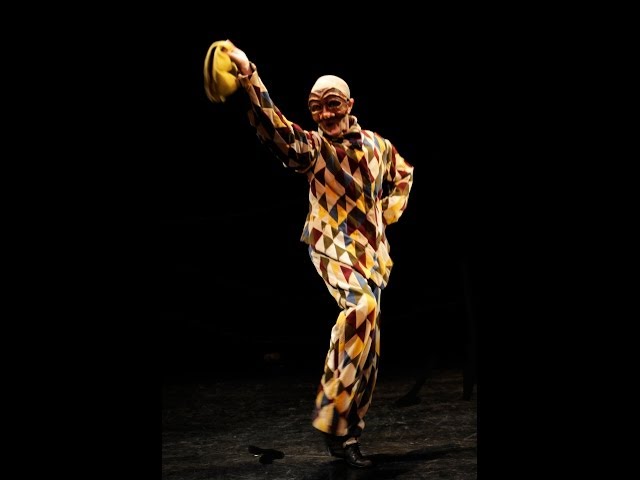The image depicts a performer in a dynamic dance pose, with a mysterious and somewhat eerie appearance. The dancer's right knee is bent and their left leg is extended, indicating movement. They are dressed in a coordinated outfit featuring a complex pattern of triangles and diamonds in colors ranging from maroon, gold, beige, red to blue, all set against a tan background. The pattern seamlessly blends from the jacket to the pants. In their right hand, the dancer holds a yellow hat while their left hand rests on their waist.

The figure’s face is concealed by a striking mask, with an unsettling look characterized by large eyes, a bald head, and exaggerated features including a pronounced nose and a possibly decorated area around the mouth that might resemble a mustache. The makeup, if present, suggests a traditional or theatrical aesthetic, possibly hinting at a French or harlequin influence with a white-painted head and red-painted face.

The scene is set against a jet-black background, creating a stark contrast that highlights the figure and their colorful attire. The floor beneath appears to be wooden, bathed in light as if from a spotlight, suggesting a stage setting and enhancing the dramatic effect of the photograph.